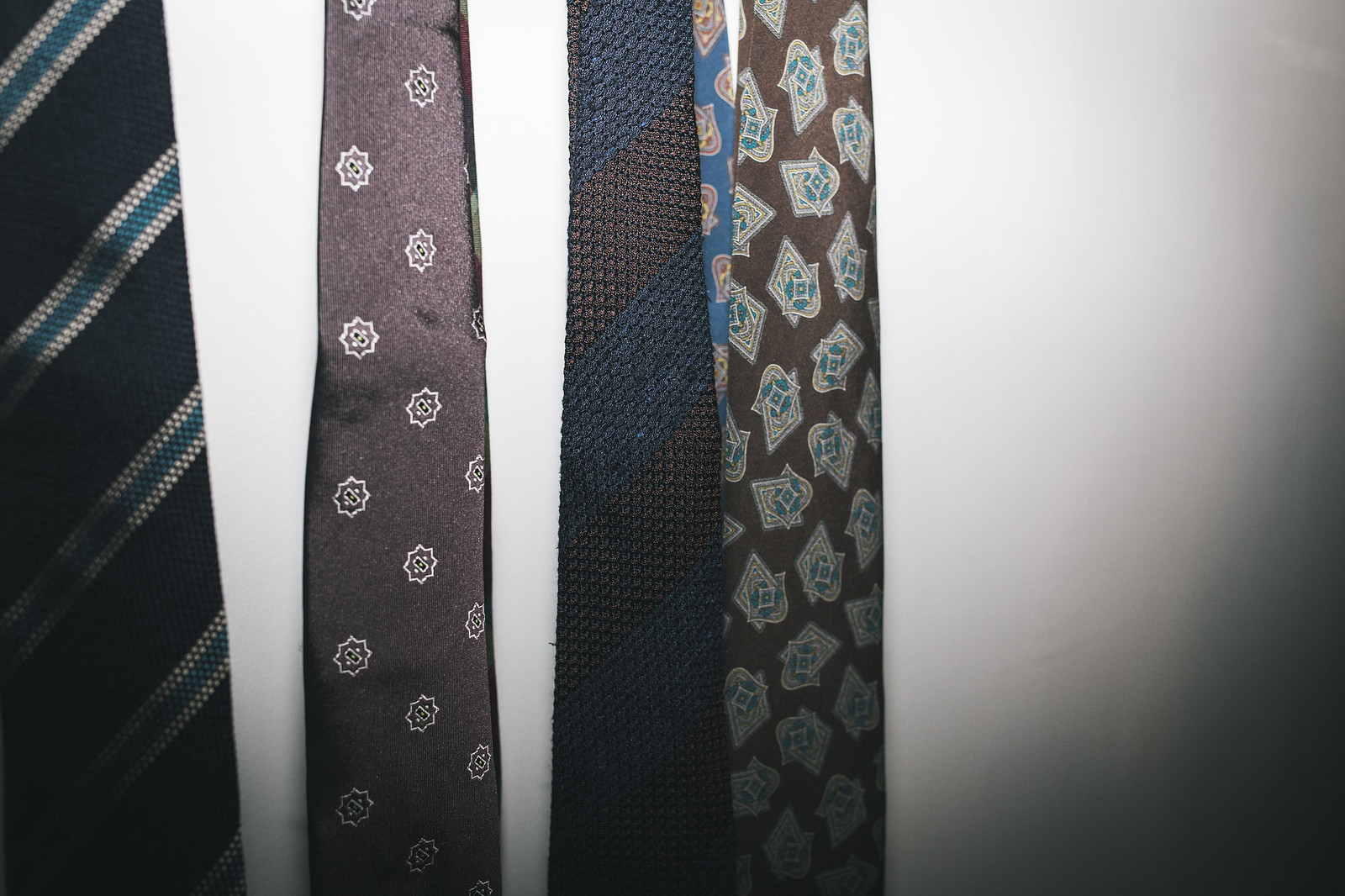This color photograph features four distinct neckties arranged horizontally against a creamy beige background that transitions into darker shadows at the bottom right. The first tie on the far left is a dark navy blue with a lighter green diagonal stripe accompanied by subtle silver patterning. The second tie is a metallic brown adorned with intricate sun-like shapes, each featuring a central star-like pattern with ten points, encased in a smaller square with dual dots at each corner. Moving right, the third tie is a dark blue and black design, with large, nearly indistinguishable diagonal stripes due to their similar tonal darkness. Finally, the tie on the far right showcases a brown geometric pattern against a base that appears metallic brown; this tie's design features geometric shapes in a goldish-gray hue.